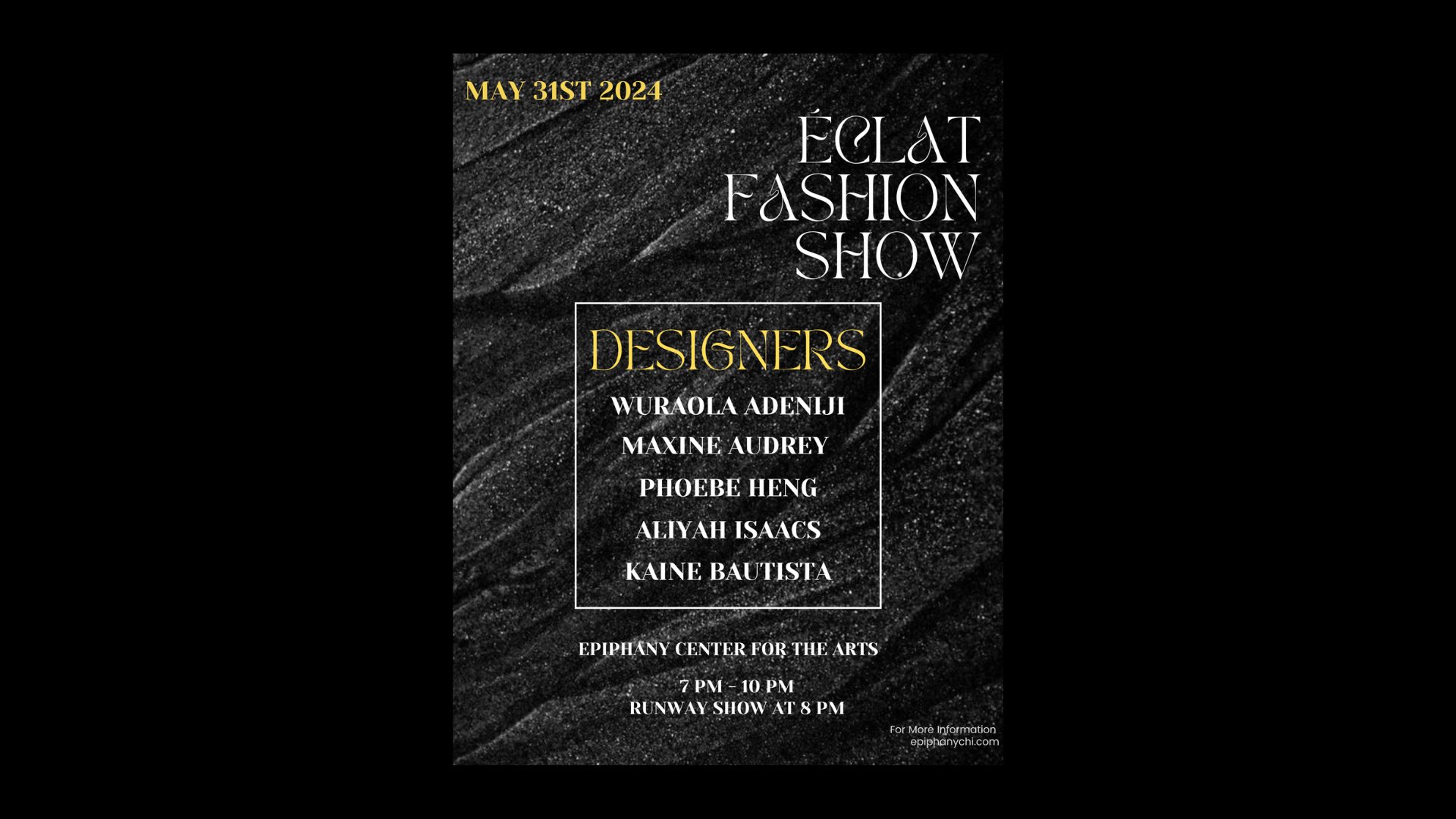The advertisement features a predominantly black background, which appears to display a close-up texture that could resemble either stone or wood, rendered in black and white. At the top left corner, the date "May 31st, 2024" is presented in a gold-colored font. Centered on the poster, the main title reads "ECLAT Fashion Show" in a stylized white shadow text. Below, encased in a box with gold lettering, the word "Designers" is prominently displayed, followed by a vertical list of names: Wu Rollo, Adenogy, Maxine Audrey, Phobie Heng, Aaliyah Isaacs, and Kane Bautista. The bottom of the advertisement states, "Epiphany Center for the Arts, 7 pm - 10 pm, Runway Show at 8 pm." There is some smaller, unreadable print located in the lower right corner.